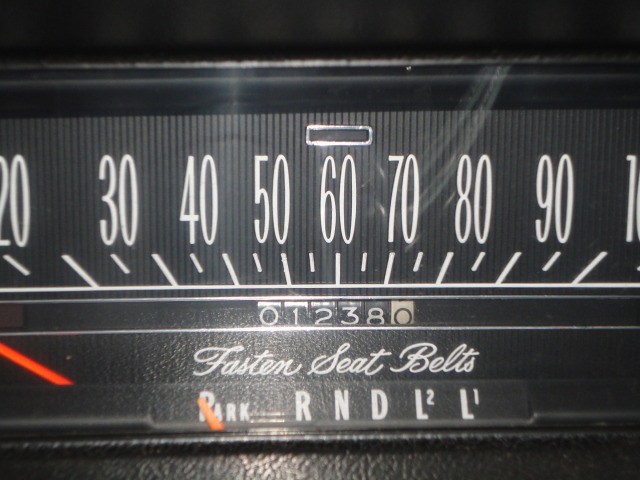Close-up of a vintage car dashboard, showcasing a unique rectangular speedometer from an old American car brand. The speedometer, reminiscent of a radio display, features white numbers and dash lines on a black ribbed background, indicating speeds from 20 to 100 in increments of 10. Below the speedometer is an odometer with turning dials displaying the numbers 01238; the last dial, indicating tenths of a mile, is inverted with a white background and black numbers. A white script beneath the odometer reads, "Fasten Seat Belts." The dashboard also includes a red indicator light, an adjacent gear display labeled "Park, R, N, D, L2, L1," and a white pointer set to "Park," implying the vehicle is stationary. This setup suggests the car might feature a three-on-the-tree column-mounted gear shifter.